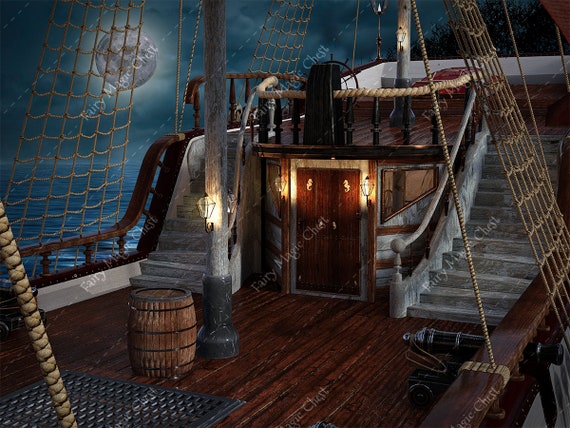This digital image, resembling a scene from a video game or CGI rendering, portrays the deck of an old wooden sailing ship, akin to a pirate vessel. The deck features a prominent wooden barrel bound by four black metal bands, positioned next to a mast with a black steel base and a tan wooden pole extending upwards. The ship is equipped with a steering wheel situated atop an upper deck, accessible via stairs on both the left and right sides. Directly below the steering wheel are two small, vertical wooden doors leading to the lower decks. The sides of the ship are lined with rigging, rope ladders that ascend to the mast, and netting, which partly obscures the full moon in the upper left corner of the image. Surrounding the deck, a wooden railing encapsulates the scene while the ocean stretches out on the left side of the ship. The night setting is accentuated by the glowing full moon, enhancing the reflective water surface. Notably, the image is overlaid with multiple slanted watermarks reading "fairy magic chest," deterring unauthorized use. The absence of any crew gives the scene a still, almost eerie ambiance.